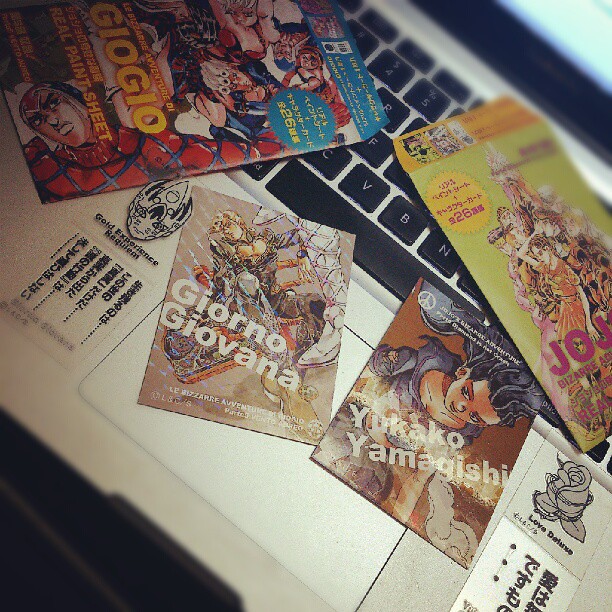The photograph provides a close-up view of a silver laptop with black keys, shot from above. Just visible at the upper edge is a portion of the laptop screen. The keyboard is littered with various colorful pieces of anime-related ephemera, creating a vibrant collage. Among the items is a comic book featuring various superheroes at the top of the image, and a series of tickets and smaller comic books beneath. One ticket prominently reads "gold experience required" and features a mask along with Asian characters. Another item displays the name "Giorno Giovanna" with an anime character wearing boots. Nearby, an item featuring "Yukako Yamagishi" depicts a character with long black hair. Additionally, there is an envelope, lime green with a yellow emblem, though its text is hard to decipher. Lastly, another ticket reads "Love Deluxe" and showcases a flower illustration. The scattered arrangement provides a visually rich and detailed scene focused on anime culture.